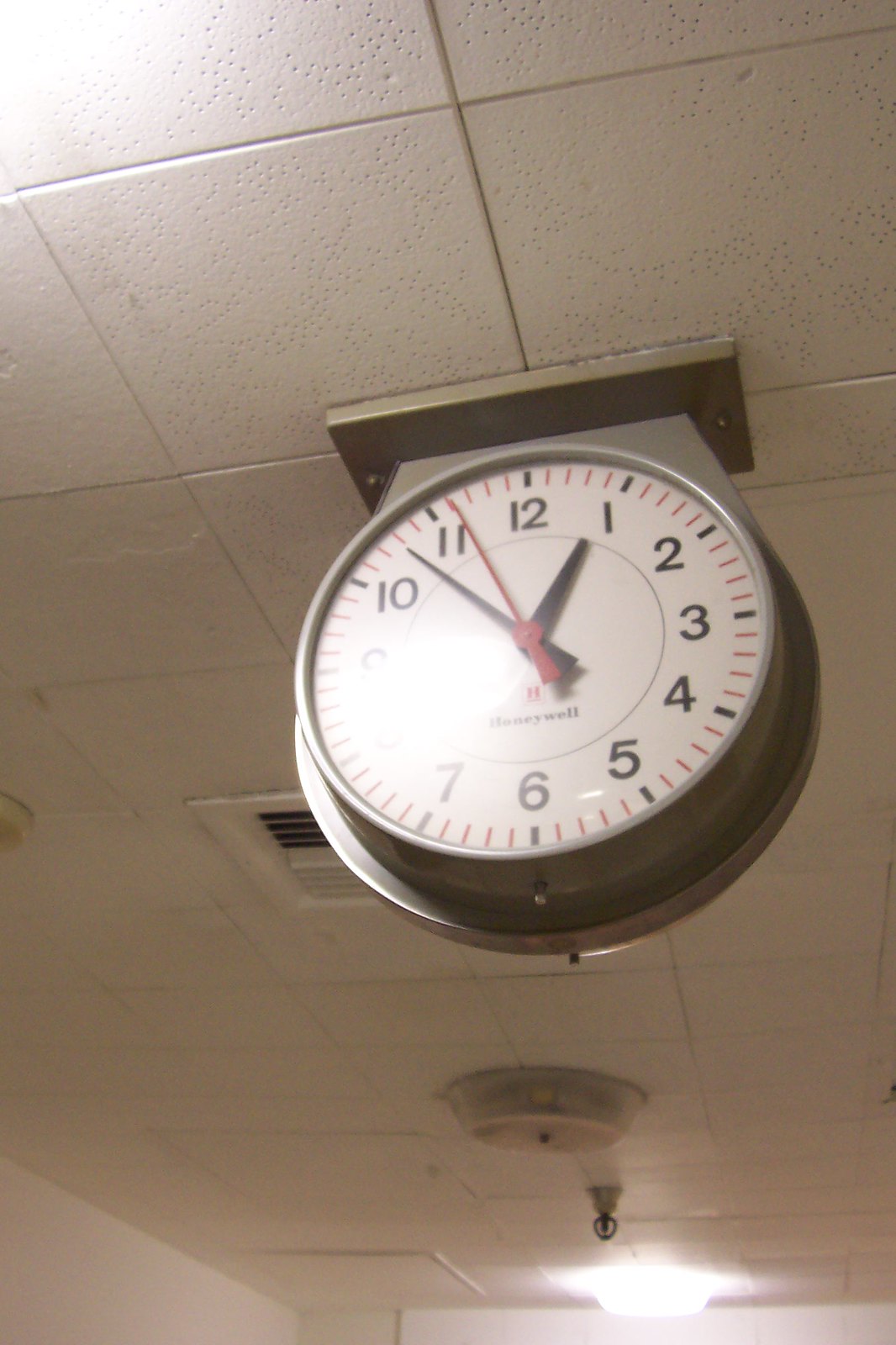In this somewhat lower resolution, vintage-style image, we observe a scene with a stark white drop ceiling, characterized by its square tiles, but tinted with a sepia tone indicating age. Centrally, affixed to the ceiling via hardware, hangs a simple silver or aluminum wall clock with a white face. The clock features bold black numbers from 1 to 12, with two black hands indicating the hour and minute, and a thin red hand marking the seconds. The time displayed is 12:53. Behind and slightly offset from the clock, a ceiling sprinkler is visible. Positioned in front of the sprinkler, we can see a round object, likely a smoke alarm. To the left of the clock, part of a ventilation grate is visible, embedded in the drop ceiling, contributing to the overall retro ambiance of the image.